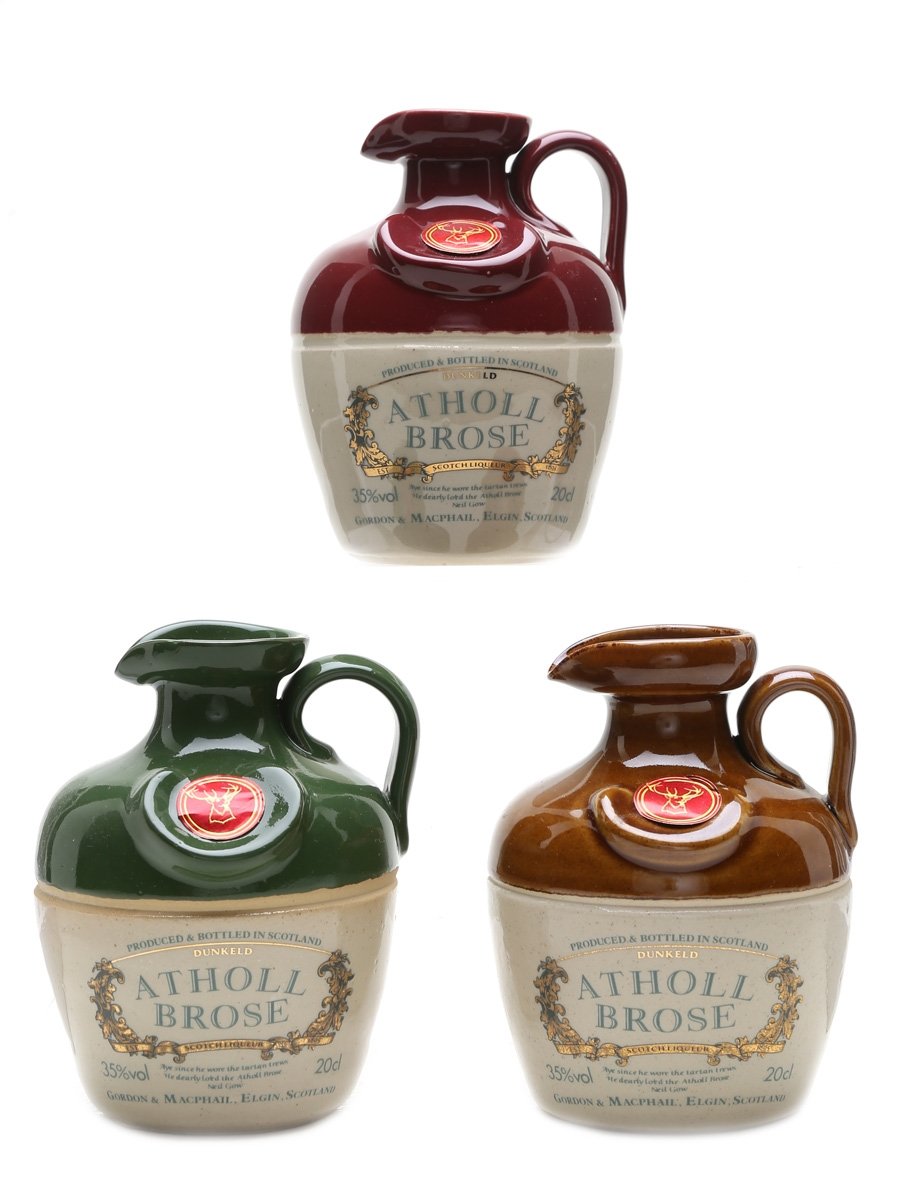The image showcases three bottles of Scotch liqueur, each produced and bottled by Athol Bros in Scotland, with a 35% alcohol by volume. The bottles are uniquely shaped, resembling a stout, teapot-like form with a small handle and short spout. Placed on a white background, they appear to have been cut and pasted into the scene rather than arranged in a single photograph. Positioned in a triangular layout, one bottle is at the top center with a reddish-purple cap, while the two at the bottom have green and brown caps respectively. All bottles share similar design elements, including the brand name Athol Bros and a distinctive deer symbol on top of each, and are oriented facing left.